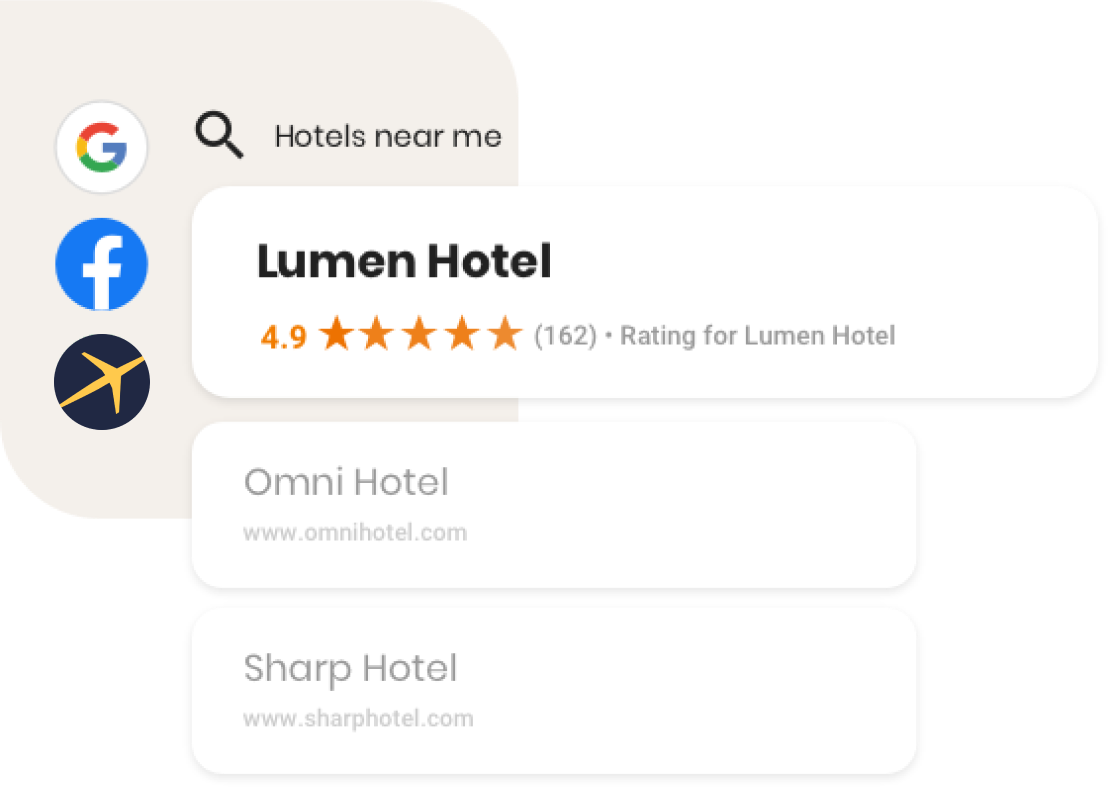Detailed Caption: 

The image appears to be a partial screenshot, potentially from a Google search. Dominating the upper portion of the image is a search bar with a magnifying glass icon, though the bar itself isn’t fully visible. Next to the icon, the search query, “hotels near me,” is shown in black text.

Directly below the search bar, there is a white rectangular box with rounded corners. Within this box, the text “Lumen Hotel” is prominently displayed in bold black letters. Just beneath this, the hotel's rating is indicated by a gold-colored "4.9" next to a series of five gold stars, signifying a near-perfect rating. Specifically, the average rating stands at 4.9 out of 5 stars. Following the star rating, “(162)” is enclosed in parentheses, highlighting that 162 reviews have been submitted for Lumen Hotel.

Below the Lumen Hotel listing, there are additional, slightly blurred boxes for other hotels such as Omni Hotel and Sharp Hotel, though these details are less clear.

To the left side of the image, three small icons are visible, representing different platforms or services: a Google icon, a Facebook icon, and an icon of a gold airplane silhouette enclosed in a purple circle, the latter of which is less identifiable.

This concise yet comprehensive layout provides essential details about Lumen Hotel's rating and review count, along with a partial view of additional hotel options and related service icons.